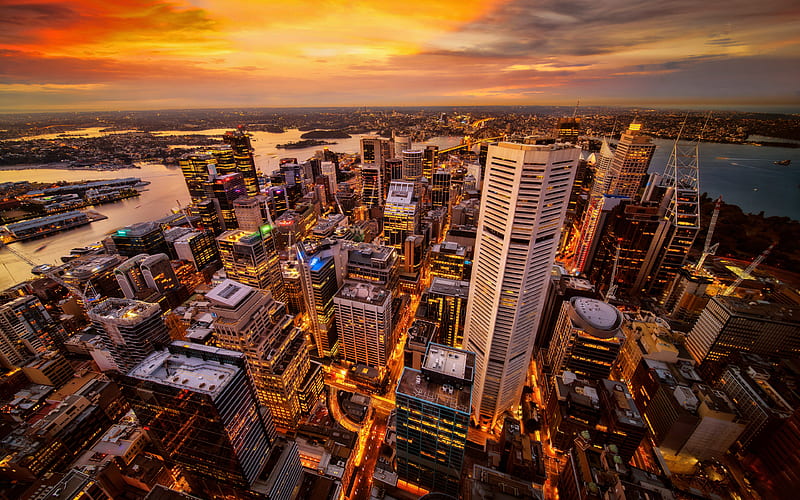This horizontal, wide-angle photograph captures a dramatic aerial view of a bustling port city's skyline at either dawn or dusk, as evidenced by the sun-kissed sky awash with vibrant red, orange, yellow, and pink hues. The city is situated on a harbor, likely surrounded by water on three sides, creating a near U-shaped formation visible from the highest vantage point. The skyline features a mix of towering skyscrapers, with the tallest building just slightly right of center, and numerous other buildings of varying heights, mostly around 10 to 20 stories. The city’s layout hints at a grid pattern, with streets far below illuminated by the yellow lights of heavy traffic, suggesting a densely populated, metropolitan area. The scene is further accentuated by the interplay of artificial and natural light, creating a stunning, almost cinematic quality.